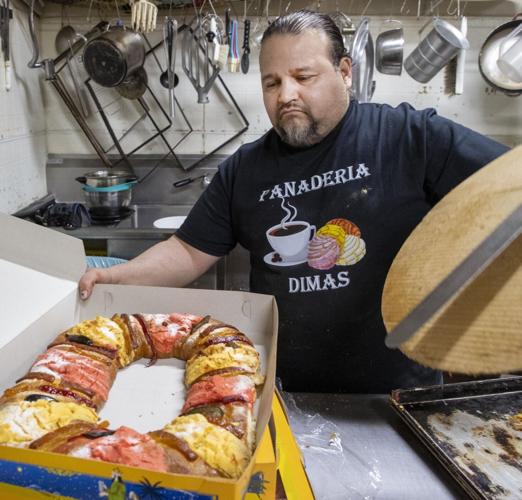In this detailed image of an industrial kitchen, a fairly large man with long, tied-up hair and a small brown and white beard is examining a large, donut-shaped pastry that alternates between yellow, brown, and pink. The pastry is contained within a cardboard box. The man is dressed in a black t-shirt that reads "Panaderia Dimas" and features a picture of a coffee mug with coffee and some pastries. He holds a serving tray with a black stripe in one hand while he looks at the pastry, possibly preparing to serve it. The background reveals a professional cooking area, with metal kitchen utensils, pots, and pans hanging on the wall, a sink behind him, and stainless steel tables equipped for cooking. A baking pan is also visible in the lower left corner of the image. The overarching colors in the image include brown, silver, red, yellow, white, and pink, contributing to a busy and functional kitchen setting.